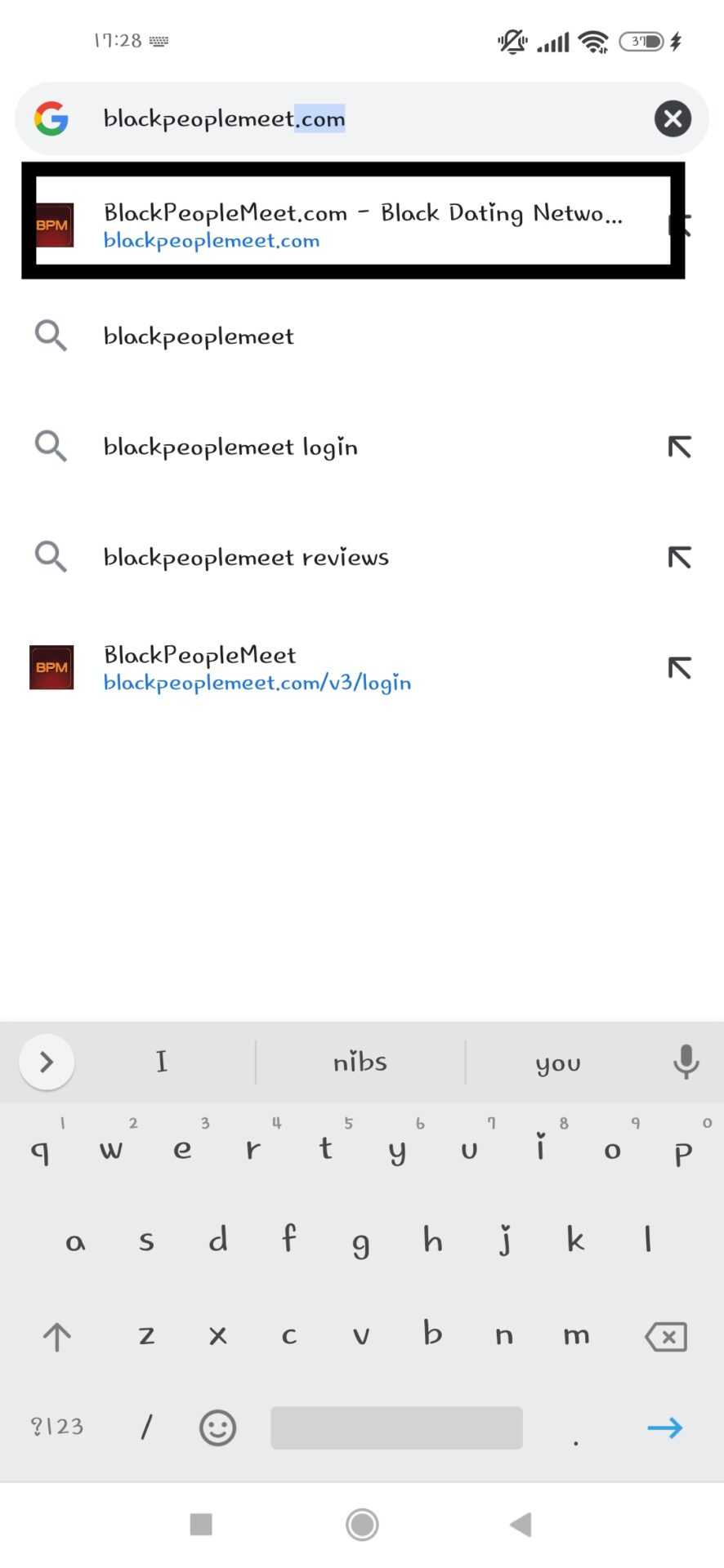The image depicts the homepage of a dating website called BlackPeopleMeet.com. The text on the page is displayed in an unconventional and somewhat difficult-to-read font, suggesting that the user may have customized their browser settings for a unique look, although it compromises readability. BlackPeopleMeet.com is a niche dating platform specifically designed for Black individuals seeking meaningful connections or relationships. Despite its specific target audience, it appears to be relatively unknown to the person describing the image. The choice of atypical typography adds an extra layer of peculiarity to the website's presentation in the browser, making it a noteworthy visual detail in the context of online dating services.